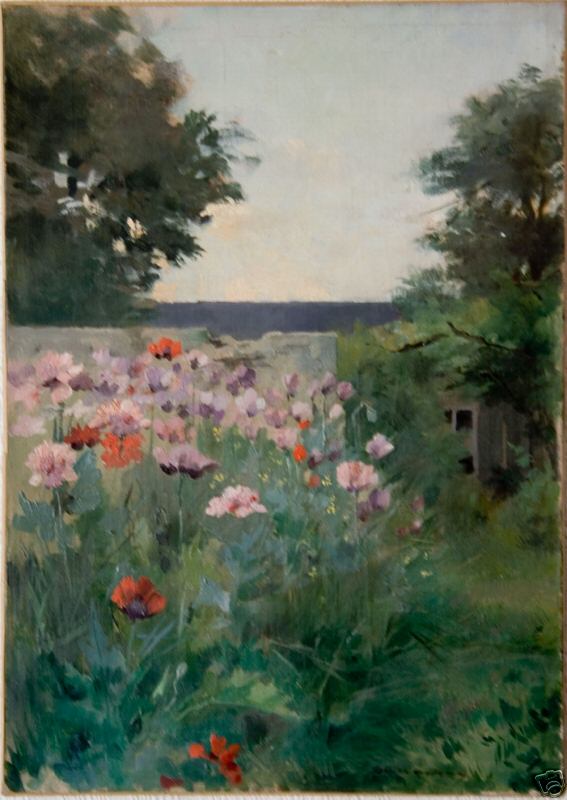This detailed and vibrant oil painting captures an outdoor rural scene with a captivating array of multicolored wildflowers growing in a lush, overgrown grassy field. The flowers, including shades of pink, orange, red, and lavender, are meticulously drawn and appear almost lifelike. They are primarily situated in the lower left quadrant of the image, blending seamlessly with the tall grass surrounding them. The background reveals an expanse of trees flanking both sides of the painting, while a distant wooden structure, possibly a house or cabin, is partially hidden behind the trees on the right. Above, the sky stretches out with a dull bluish-gray hue and scattered white clouds, suggesting it is daylight. There are also hints of gray, which might indicate the presence of a body of water under the skyline, adding to the scene's tranquil atmosphere. Decorative elements such as possible cinder blocks or rocks add subtle complexity to the foreground. The overall composition exudes a peaceful, rustic charm, making it an ideal piece for a cozy home entryway or dining room.